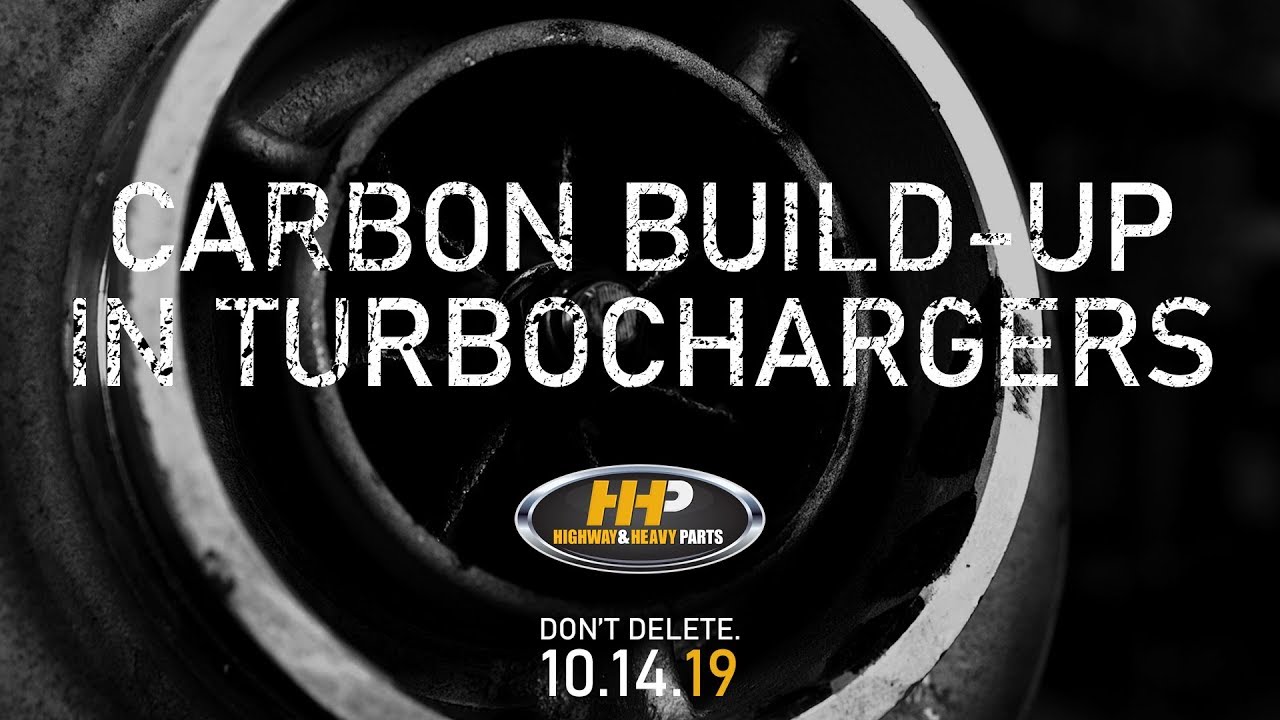The black-and-white image appears to be an advertisement aimed at car enthusiasts, specifically addressing the issue of carbon buildup in turbochargers. Central to the image are bold, white, capitalized letters stating "CARBON BUILDUP IN TURBOCHARGERS." The text has a worn, textured appearance, adding a rugged feel. Behind this text lies a partially visible metallic object, likely a turbocharger, rendered in shades of silver, black, and gray. Below the main text, there's an oval logo reading "HHP" in yellow letters, followed by "Highway and Heavy Parts." Further down, in white capitalized letters, the phrase "DON'T DELETE" is prominently displayed, with the date "10.14.19" beneath it, where the "19" is highlighted in yellow. The overall image is sharply defined, with a clear and bright setting that suggests natural lighting.